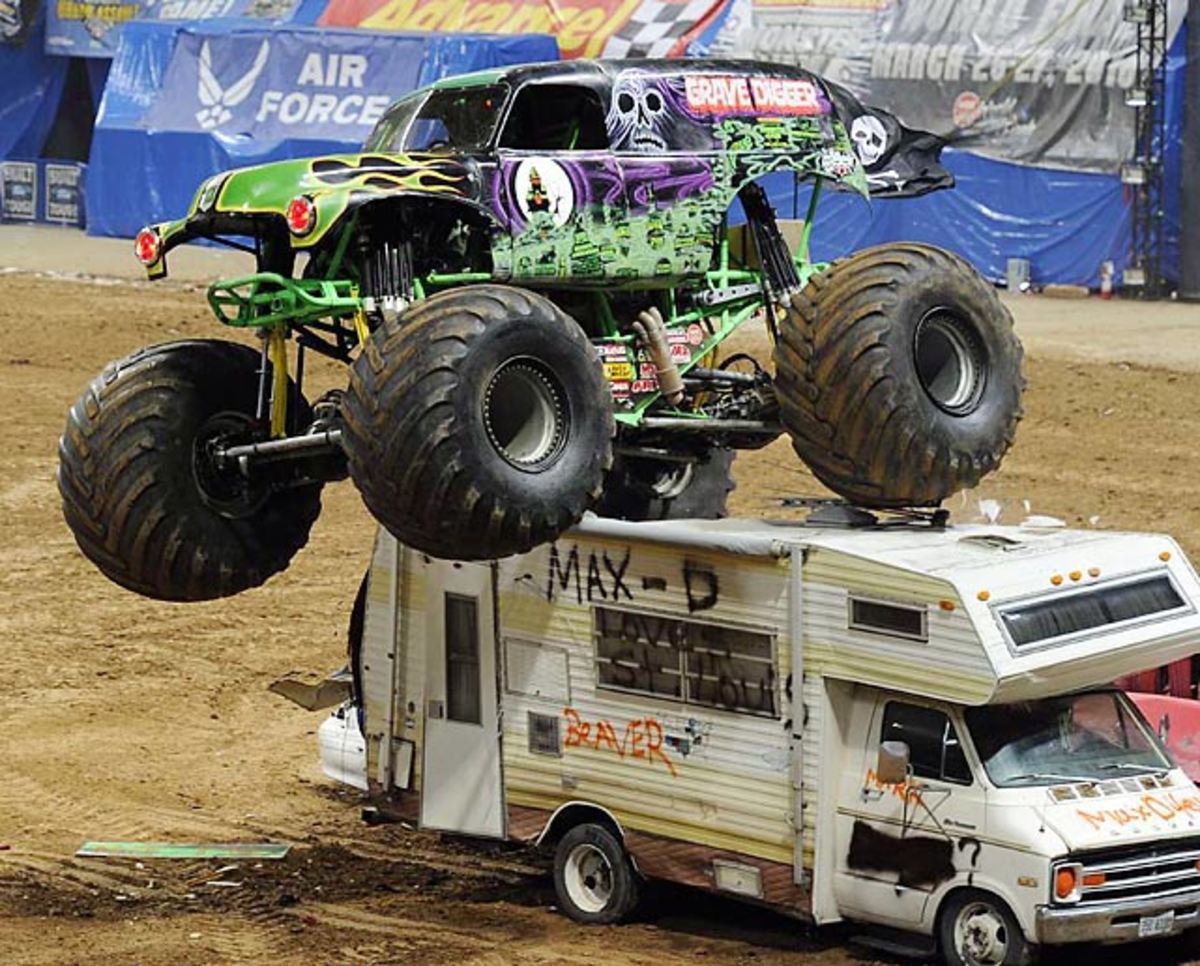This vibrant photograph captures an exhilarating moment at a monster truck show, featuring a massive green and purple monster truck named Grave Digger in mid-air above a crushed white camper van that bears the name "Max D. Braver." The monstrous vehicle, adorned with ghostly skeletons and green flames, boasts gigantic, mud-covered tires, with one of them crushing the roof of the RV while the others hover above. The stadium's dirt-covered ground sets the stage for this dramatic scene, with a blue barrier in the background displaying an advertisement for the Air Force, partly obscured by tarps. The sheer energy and chaos of the monster truck soaring over the damaged RV are vividly captured, reflecting the thrilling atmosphere of the event.